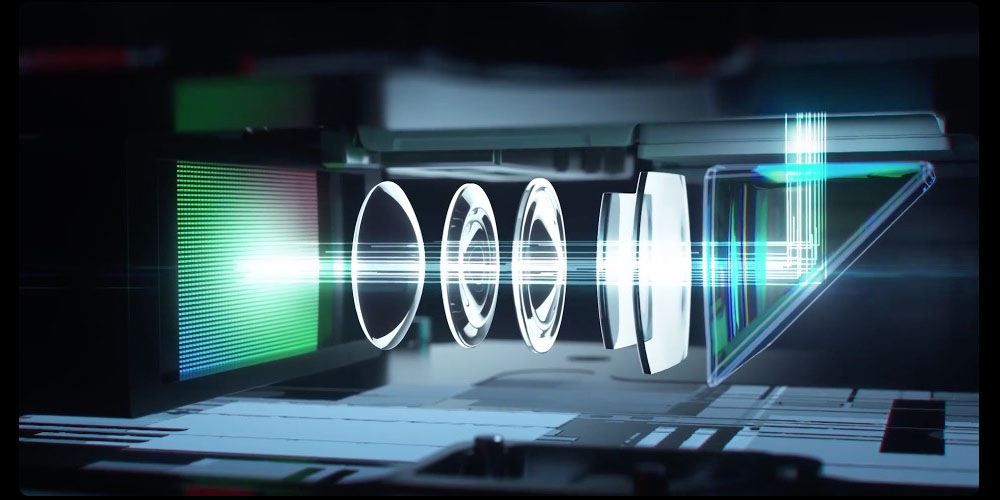The image presents a digital artwork resembling a sophisticated recording studio or computer workstation. Dominating the left side of the frame is a green screen set at an angle against a black background, featuring horizontal lines receding into the distance. A streak of light extends horizontally from the center of this screen, passing through three white circles with brighter interiors before traversing two rectangular glass-like objects. It then makes contact with a blue-bordered triangle, which redirects the light upwards into a white area at the top. The scene is enhanced by the presence of green, blue, red, and pink hues emanating from the screen, lending it a vibrant and dynamic atmosphere. The bottom of the image is white, adding to the bright and clear setting, while the overall composition, lacking any textual or numerical elements, highlights the sleek and meticulously designed, possibly computer-generated, aesthetic of a high-tech studio or workstation.